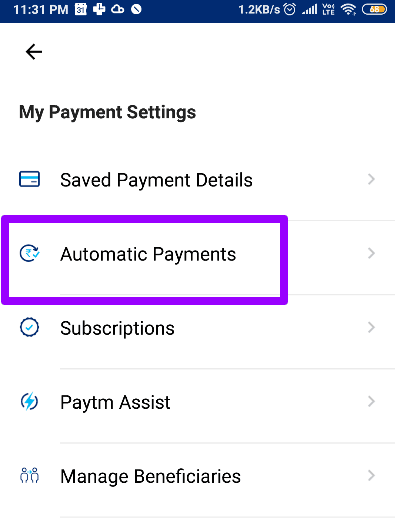This screenshot, captured from an unspecified mobile device, displays a user interface characterized by several elements identifiable at the top of the screen. On the top left corner, the time is indicated as 11:31 PM, accompanied by several notification icons, including a calendar notification, an icon resembling a cross with clock hands, a cloud storage notification, and a circle crossed diagonally. On the top right corner, additional indicators include a data transfer rate of 1.2 kB per second, a timer icon, a mobile data icon, a VOLTE icon, a WiFi signal icon, and a battery level showing 68%.

The main content of the screen features a heading titled "My Payment Settings." Under this heading, there are five clickable sections listed vertically: "Saved Payment Details," "Automatic Payments," "Subscriptions," "PAYTM Assist," and "Managed Beneficiaries." Each section is accompanied by a small icon on its left and rightward-pointing arrows for expansion on the right. Notably, the "Automatic Payments" section is highlighted by a bright, neon-purple rectangular outline, indicating post-screenshot editing. The overall design of the interface is clean and minimalist, with a white background and blue accents throughout.